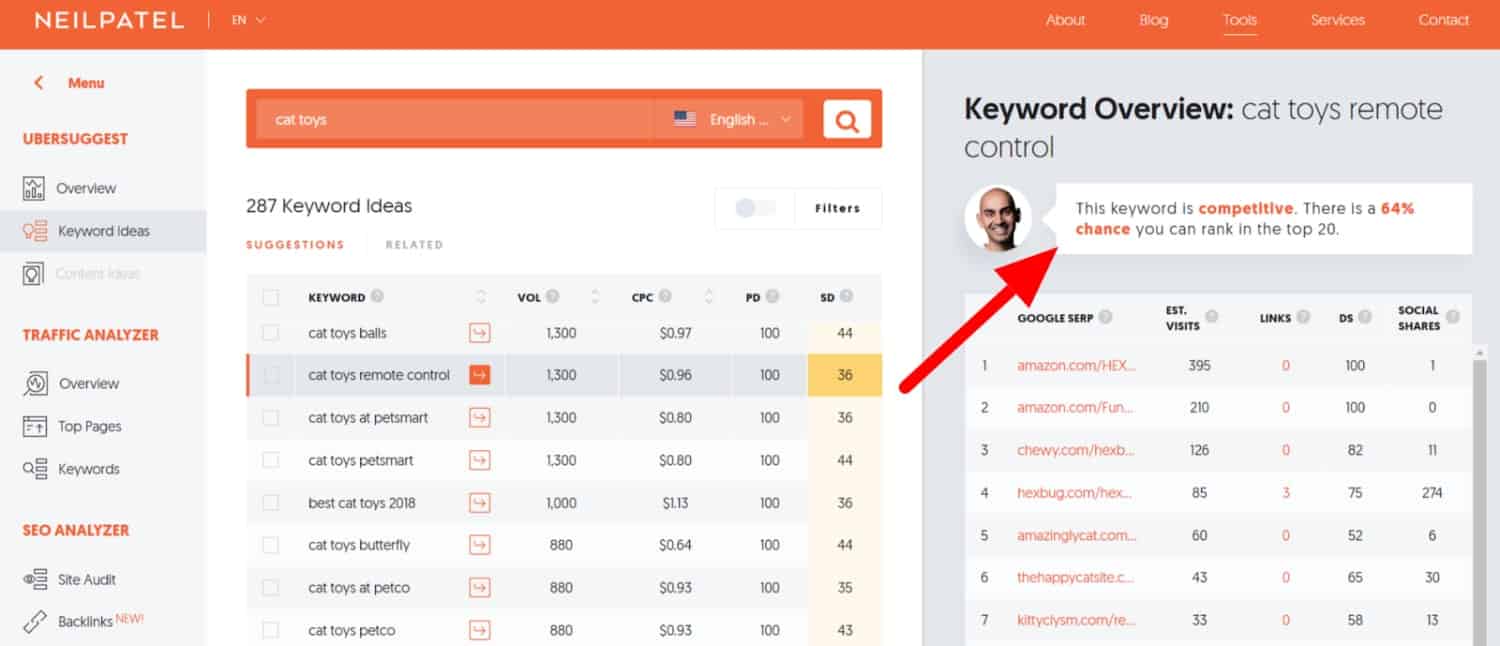In this image, several menu sections are presented against a predominantly white background, with some gray accents and a striking use of orange. On the left side, an orange-colored vertical sidebar features a long list of options, starting with "Neil Patel" at the top. Below this, the options span downwards and include categories such as "Home," "Blog," "Tools," "Services," and "Content."

Moving centrally, there is a dropdown menu displaying various tools for website optimization. The options listed are "Ubersuggest," "Overview," "Keyword Ideas," "Traffic Analyzer," "Overview," "Top Pages," "Keywords," and "SEO Analyzer," which further breaks down into "Site Audit" and "Backlinks."

At the center of the image, there's a gray-background section featuring a search bar at the top followed by a list titled "267 Keyword Ideas." This list appears to be tools intended for keyword research, likely aimed at optimizing a website for search engines. The keywords, related mainly to toys, include terms like "cat toys," "cat toys remote control," "butterfly cat toys," and "Petco," each with associated pricing details.

To the right side of the image, there is another box with a library-like background where URLs are listed. At the top of this section, there's a portrait of a man with a caption indicating that a particular keyword is competitive and suggests the possibility of ranking within the top 20 results. Below this, additional suggested keywords and numeric data are provided to help enhance the website's content and marketing strategy.